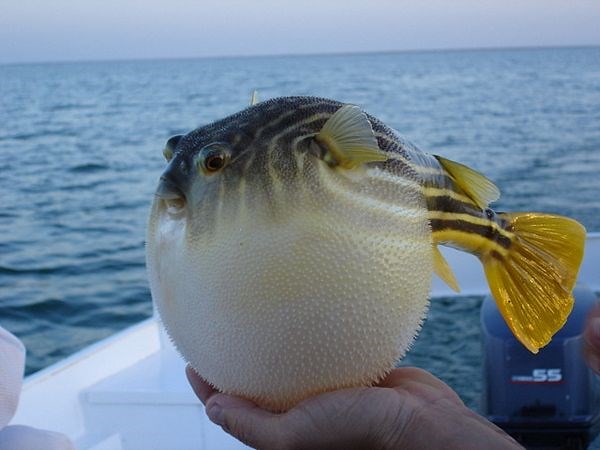In this photograph taken from a white boat against a backdrop of blue ocean and a light blue, slightly cloudy sky, a person holds a distinctively round, puffed-up puffer fish. The fish's top is patterned with black stripes and yellow hues, culminating in bright golden fins near its back. The bottom portion of the fish is stark white and adorned with small spikes or hairs. Its face features prominent eyes and a mouth, with noticeable fins near the head. An additional detail visible is a black motor labeled with the number "55" situated in the bottom right of the image.